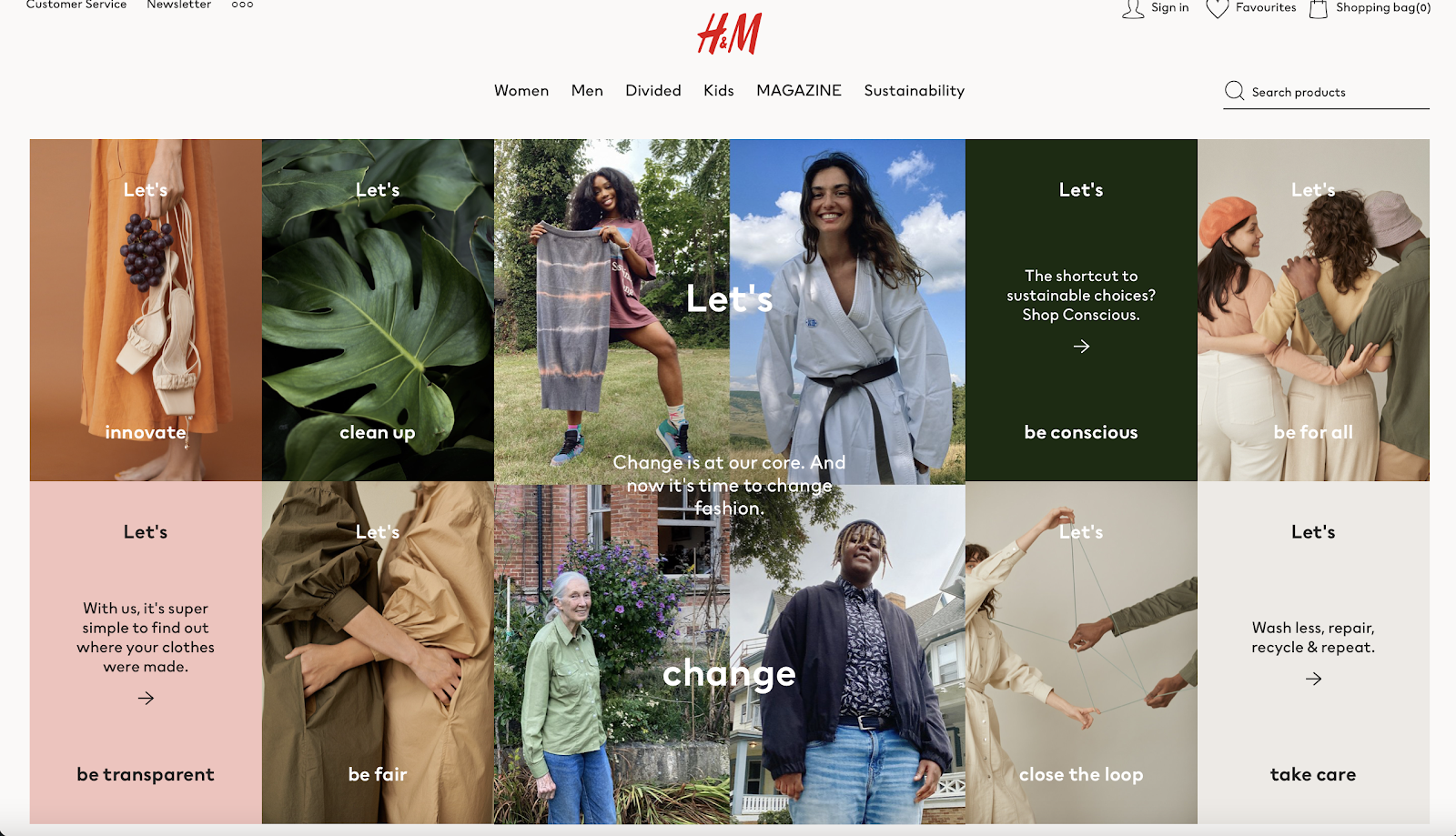A detailed screenshot of the H&M website captures a clean, modern layout starting with a light gray top border and a white page background. At the center top, the bold red H&M logo is prominently displayed, with a black navigational menu directly below listing categories: WOMEN, MEN, DIVIDED, KIDS, MAGAZINE (in all caps), and SUSTAINABILITY. On the top left-hand corner, in black text, are options for CUSTOMER SERVICE, NEWSLETTER, and three circles indicating additional features. The top right corner features SIGN IN with a profile icon, FAVORITE with a heart icon, and SHOPPING BAG with a corresponding icon.

Directly below, a search bar with the label “SEARCH PRODUCTS” is underlined and accompanied by a magnifying glass icon. The main header image is composed of a collage featuring six tall rectangular photos in a 3x3 grid layout. 

**Top Row:**
1. An orange box showing a woman in an orange dress holding beige strappy sandals and a bunch of purple grapes, standing barefoot against an orange backdrop, captioned "Let's Innovate" in white text.
2. Close-up of large green leaves with the caption "Let’s Clean Up."
3. A black woman with voluminous shoulder-length curly hair, in a maroon oversized shirt holding a gray striped towel, standing on grass with trees behind her, one knee bent.
4. A white woman with brown curly hair wearing a white taekwondo outfit outdoors against a cloudy sky.
5. A dark green box with the caption "Let’s Be Conscious," featuring text, "The Shortcut to Sustainable Choices, Shop Conscious" and a right-pointing arrow.
6. A tan-beige background featuring three individuals linked arm-in-arm: a woman with long brown hair, a curly-haired woman, and a black man in a purple bucket hat viewed from the back.

**Second Row:**
1. A light pink rectangle with the words "Let's Be Transparent" and the message "With Us, It’s Super Simple To Find Out Where Your Clothes Were Made" with a right-pointing arrow.
2. Two women in poofy raincoats, one brown and one tan, embracing with arms in each other's pockets, captioned "Let’s Be Fair."
3. An elderly woman with white hair in a low ponytail, wearing a green button-down shirt and blue jeans, standing outdoors in front of a brick house with green-leafed and purple-flowering bushes.
4. A black man with short blonde dreadlocks, wearing a patterned blue button-down shirt, jeans, and a blue jacket.
5. A gray box showing two people, one in a white dress and one with green sleeves, playing cat's cradle, captioned "Let’s Close The Loop."
6. A light gray box with black text, "Let’s Take Care," promoting washing less, repairing, recycling, and repeating, and featuring a right-pointing arrow.

Across the top four images, centered, in white text, are the words "Let’s Change." In the center of the image grid, the motivational text reads, "Change Is At Our Core And Now It’s Time to Change Fashion."